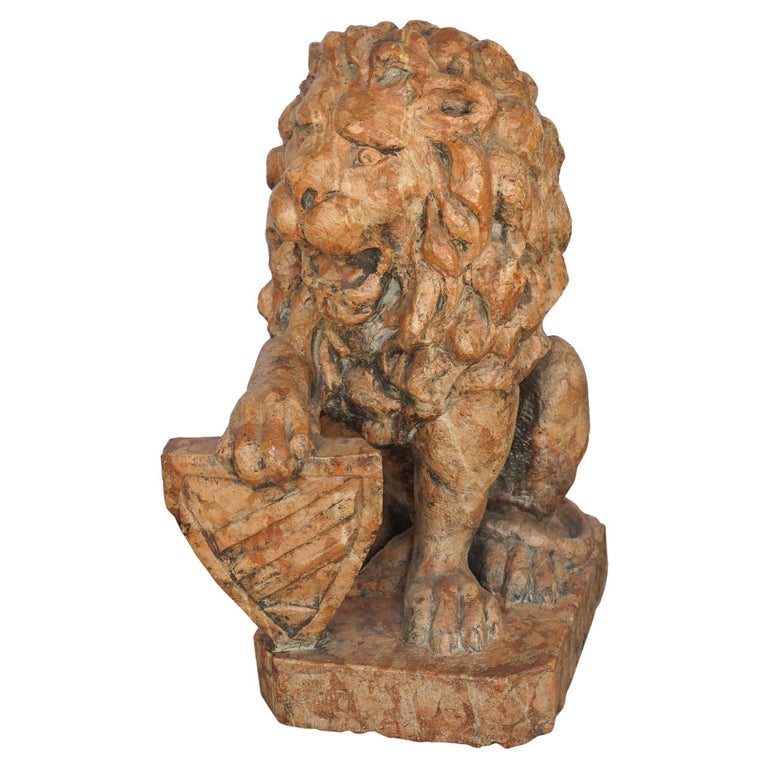The image showcases a detailed photograph of a small, intricately carved sculpture of a lion, prominently displayed against an all-white backdrop. This artistic piece is approximately five inches high and three inches wide at its broadest point, narrowing to about two inches elsewhere. The sculpture appears to be made out of either clay, rock, or wood, exhibiting a brown hue with reddish tones and blackened accents that highlight its carved details, resembling either black varnish or age-induced smudges.

The lion is depicted in a poised and majestic stance, seated on its hind legs with its left paw flat on the ground and its right paw resting on a shield. The shield, characterized by diagonal stripes running from the lower left to the upper right, has a flat top and tapers to a point at the bottom, adding to the regality of the piece. The lion's head is turned to the left, presenting a three-quarter profile so that only the left eye is visible. Despite the mouth being open as if caught mid-roar, no teeth are visible. The mane is meticulously carved in wavy patterns, enhancing the lion's noble appearance. The entire figure is raised on a rectangular pedestal, about half an inch high, serving as a solid base for this impressive piece of sculpted art.